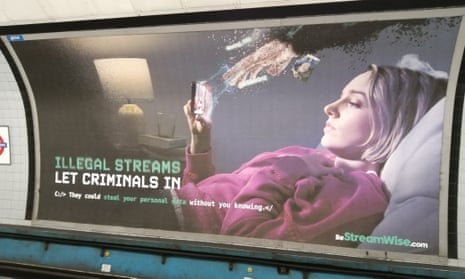The image depicts a large advertisement poster in a subway setting, identified by the curved, tunnel-like structure and a rusted, dirty blue wall beneath the billboard. The poster features a photograph of a blonde woman lounging in bed on a pillow, looking intently at a cell phone in her right hand. She wears a pink top and appears to be Caucasian. From her phone, holographic dots seem to emanate, adding a dynamic element to the image. Positioned centrally, the woman is just slightly to the right.

To the left of the woman’s image, the billboard prominently displays a Public Service Announcement (PSA) warning against illegal streaming. The bold text in green reads "ILLEGAL STREAMS" followed by "LET CRIMINALS IN" in white. Beneath this warning, in smaller, less readable text, it states that illegal streams could lead to personal data theft without the user's knowledge. The advertisement concludes with the website "streamwise.com" positioned at the bottom right.

Additional details in the image include a table lamp and an alarm clock positioned behind and to the left of the woman, along with a glass placed on top of a book, contributing to the homely yet cautionary atmosphere conveyed by the PSA.